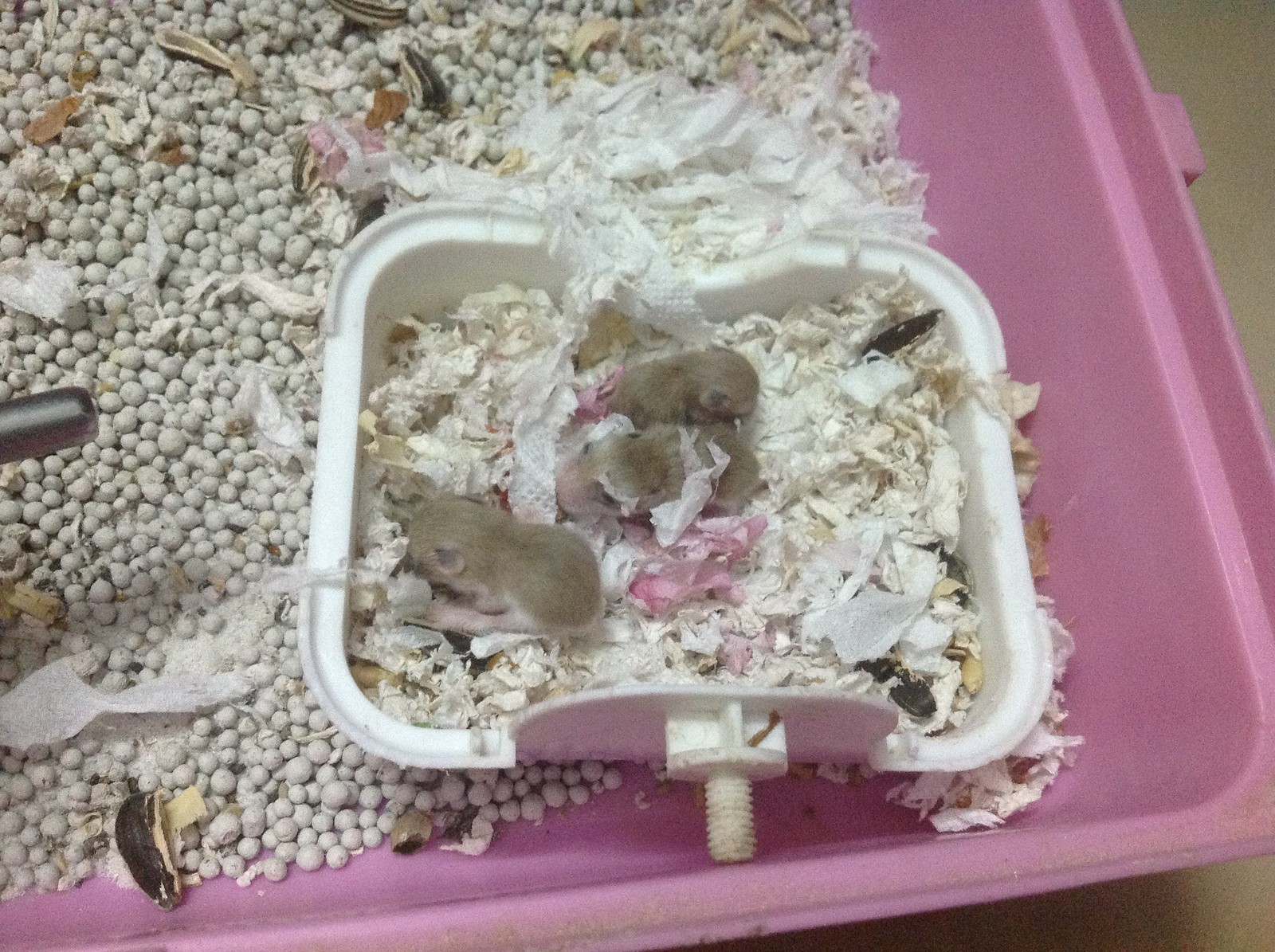This is a close-up image showcasing a corner of a pink pet rodent pen. Inside the larger pink container, there is a smaller white square bowl filled with torn-up toilet paper and newspaper serving as bedding. Nestled in the bedding are three small baby rodents, brown in color, presumably rats or mice. These babies, each about two to three times the size of sunflower seed shells scattered around, are either sleeping or resting comfortably. The floor of the pink container is also covered with similar bedding and what appears to be small white beads. To one side, the tip of a water bottle is visible, suggesting this is part of a larger cage setup for rodents.